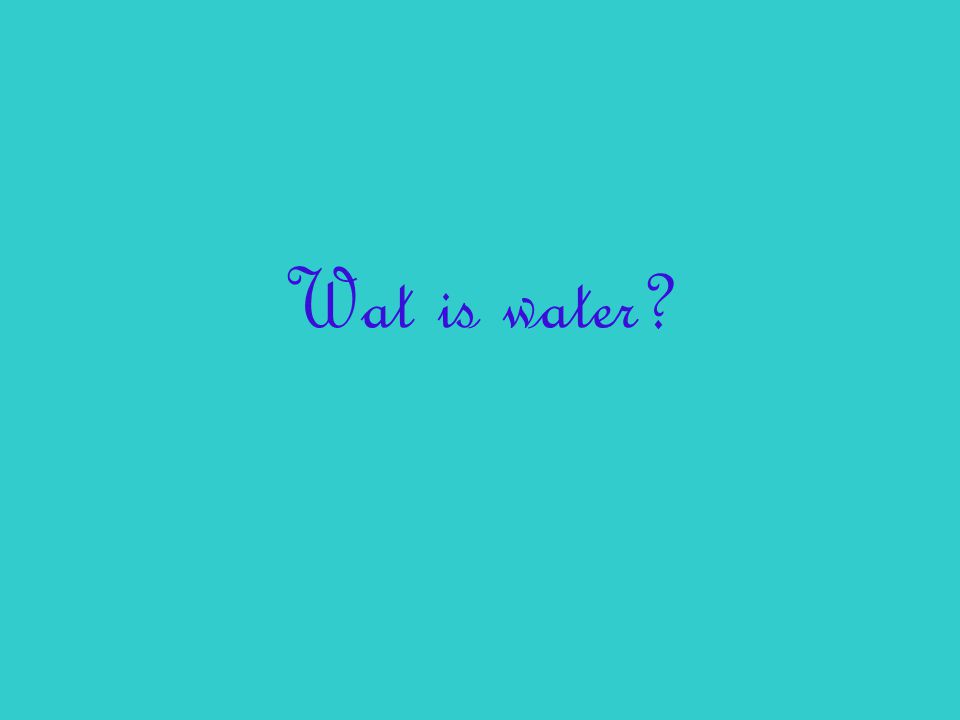The image features a strikingly vibrant teal background with a playful and feminine French cursive font that reads "WAT is water?" The text is prominently displayed in a bright, vibrant blue color, standing out crisply against the solid teal backdrop. Notably, the word "what" is misspelled as "WAT," adding a quirky element to the image. The eye is immediately drawn to the simplicity and centrality of this single question, which is perfectly centered in the middle of the square composition. The overall effect is minimalist, yet the vivid colors and elegant, curly font imbue the image with a whimsical and captivating charm.